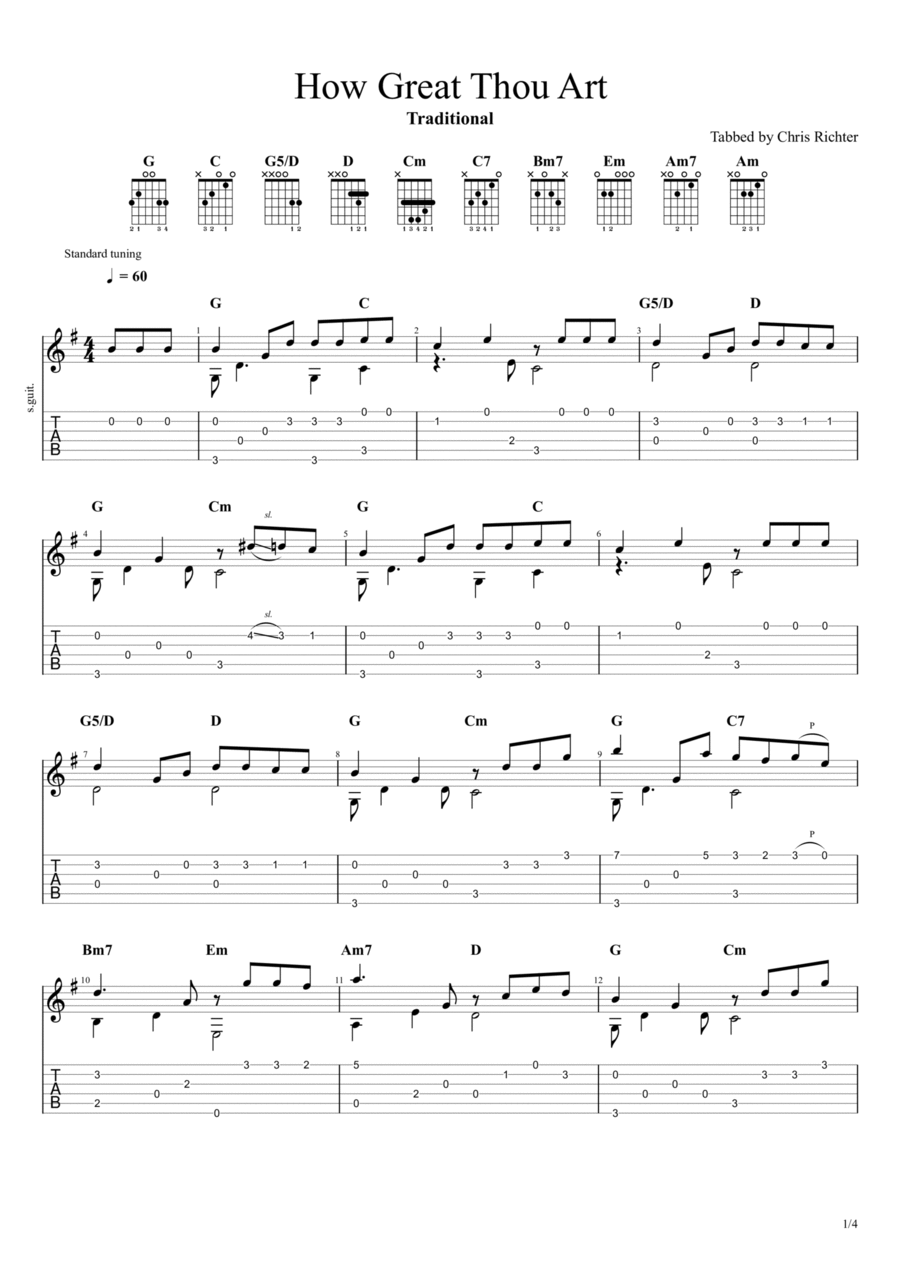This image displays a black-and-white sheet of music for the hymn "How Great Thou Art." At the top, the title "How Great Thou Art" is prominently displayed in large text, with the word "Traditional" immediately below it in smaller font. To the right, it credits Chris Richter as the person who tabbed the music. The sheet features four bars of music, which includes the standard musical notation alongside guitar tabs.

In the upper portion of the page, there's a guide that lists the coordinating notes and chords to be played. These include G, C, G5/D, D, C7, Bm7, Em, Am7, and Am. The notation indicates standard tuning with a tempo marking of a quarter note equaling 60 beats per minute. Beneath this guide are the four lines of music, set in 4/4 time with an F-sharp key signature. These lines incorporate both the treble clef notation for the melody and a separate tab section showing the specific strings to pluck and where to place fingers on the guitar.

Overall, the sheet music provides a detailed and functional layout that caters to both traditional sheet music reading and guitar tab players, making it accessible for musicians at various skill levels to play this classic hymn.